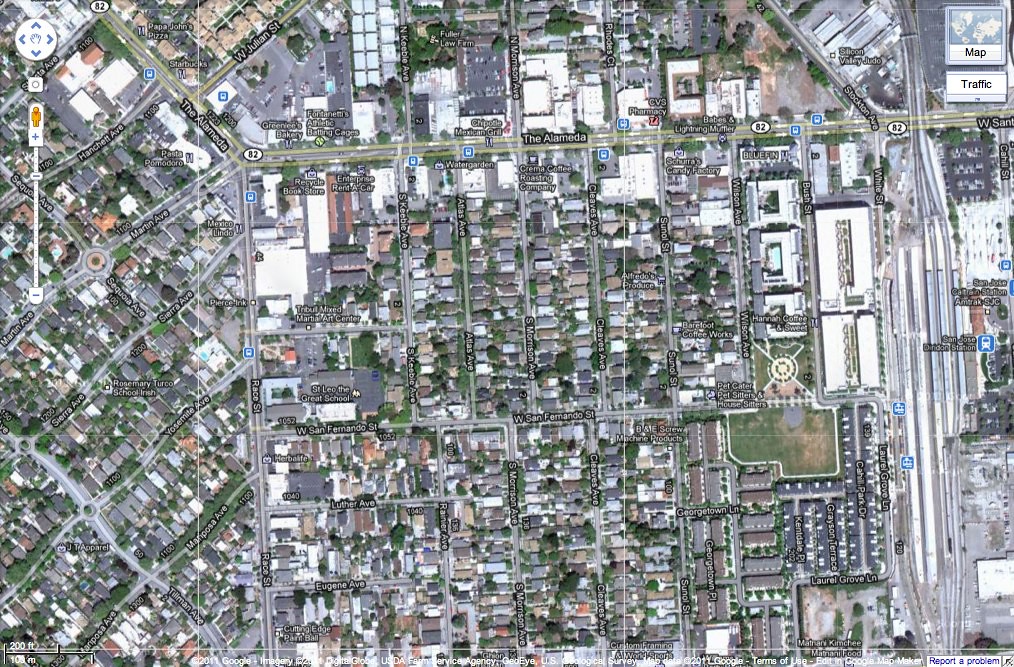This image is an overhead view of a city, resembling a Google Maps interface. In the upper left-hand corner, you can see a hand icon for dragging and moving the map, situated just above a zoom gauge for adjusting the view. In the upper right-hand corner, there's a small legend with options labeled "Map" and "Traffic." The cityscape reveals numerous houses; the high altitude of the image makes it challenging to discern specific details about the homes beyond the color of their roofs. The layout of the city varies: one section features a regular grid pattern with parallel streets, while to the left, the streets are more curvilinear, including some roundabouts. Additionally, there are visible commercial areas and possibly a train station on the far right side of the map.